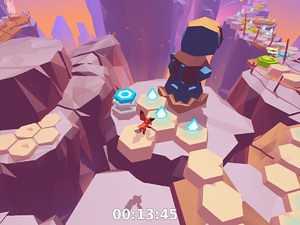The image depicts a brightly colored, cartoonish digital game featuring an anthropomorphic fox character with an orange body, black-tipped ears, and a white bushy tail. The game environment showcases a series of hexagonal platforms resembling honeycomb, forming paths that meander across vibrant, flat-topped cliffs and mountains. The cliffs exhibit a gradient of colors, transitioning from purples and pinks in the distance to browns and oranges in the foreground, enhancing the whimsical, artistic aesthetic of the scenery.

Notably, the fox is seen navigating these honeycomb-like platforms, which vary in thickness and create a stepped appearance akin to a beehive. The overall visual style uses a palette of pinks, yellows, blues, greens, and browns, exuding a kid-friendly and inviting atmosphere. In the lower part of the image, a timer reads "00:13:45," indicating the elapsed game time. The game is presented from a top-side view that highlights the winding paths and distant course ahead, potentially leading to a village or castle nestled atop the colorful cliffs. Scattered throughout the scene are distinctive turquoise and white flame elements, hinting at in-game collectibles or objectives.